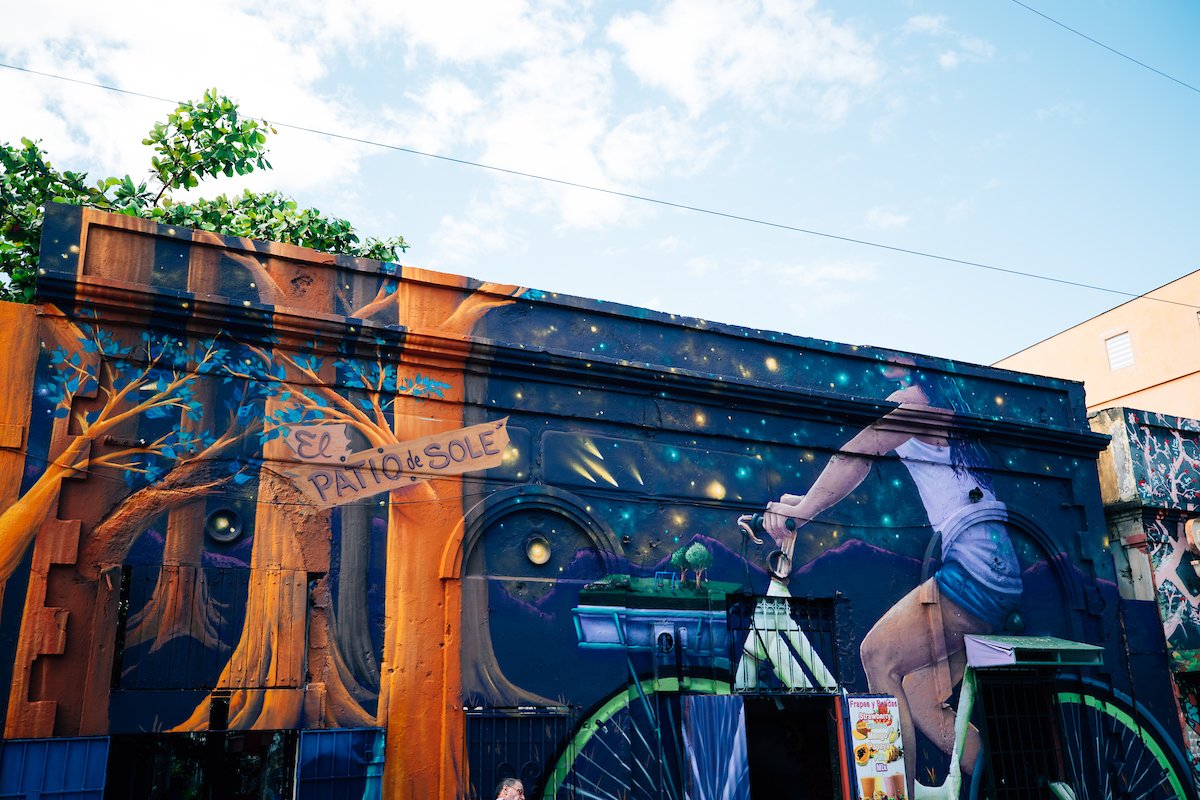The side of the building features a vibrant graffiti artwork. On the left third of the mural, five tree trunks are depicted with varying degrees of proximity. The closest tree trunk, notable for its orange hue, has two signs attached: the upper sign reads "L-E-L," and the lower sign says "Patio de Sole." The central third of the mural showcases a visually striking decorative sky filled with blue and yellow dots, some resembling comets shooting through the atmosphere. Beneath this celestial display, a series of mountain ridges are illustrated, grounding the scene. The right third of the mural, along with the bottom part of the central third, portrays a woman riding a green bicycle. Her head is not visible, as her hair seamlessly blends into the starry sky. She is dressed in a white tank top and blue shorts, adding a touch of realism to the fantastical elements of the artwork.